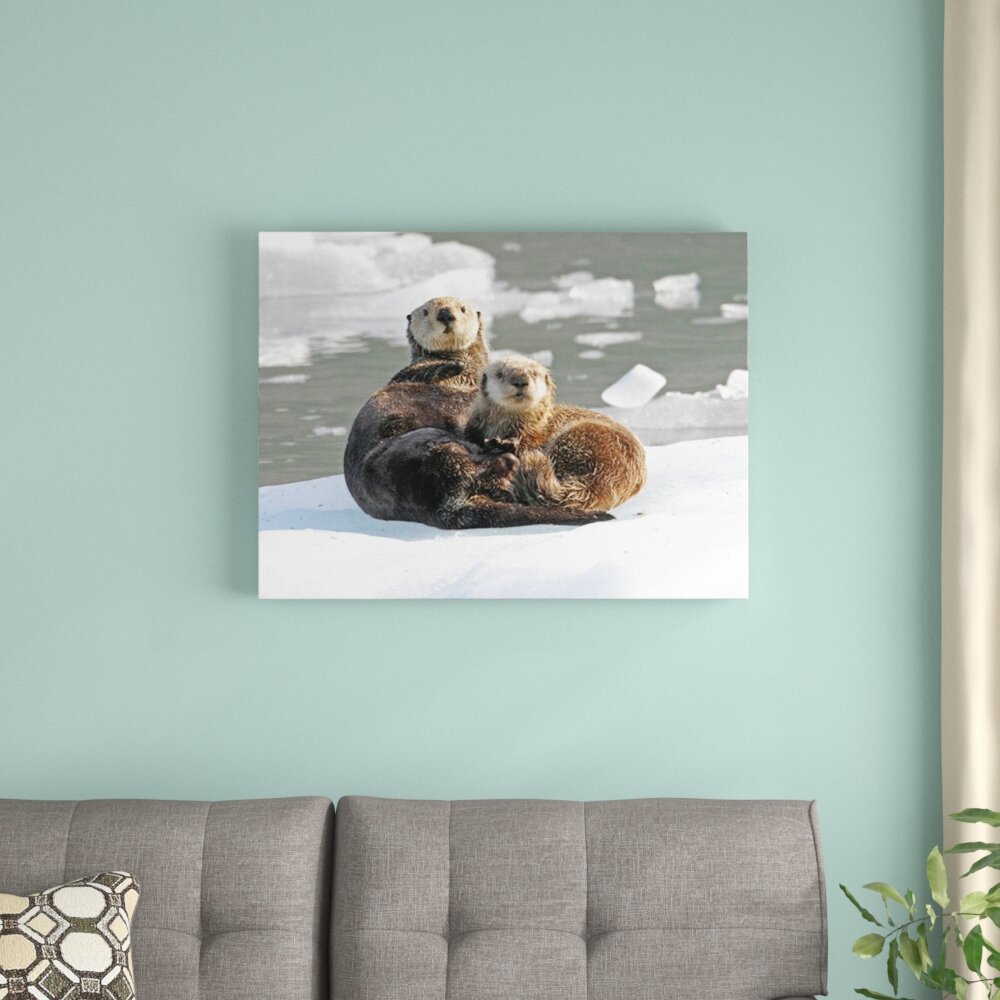This is an interior photograph showcasing a cozy room with a mint green wall. The focal point is a large rectangular photograph of two otters huddled together on a glacier, with water and ice in the background. The otters are looking directly at the viewer. Below the artwork, there is a gray sofa adorned with a decorative pillow featuring a hexagonal pattern with yellow, white, and gray spots. To the right, a green plant's branches are visible, adding a touch of nature. Along the far right edge is a white vertical column, possibly a curtain, enhancing the room's serene and artistic ambiance.